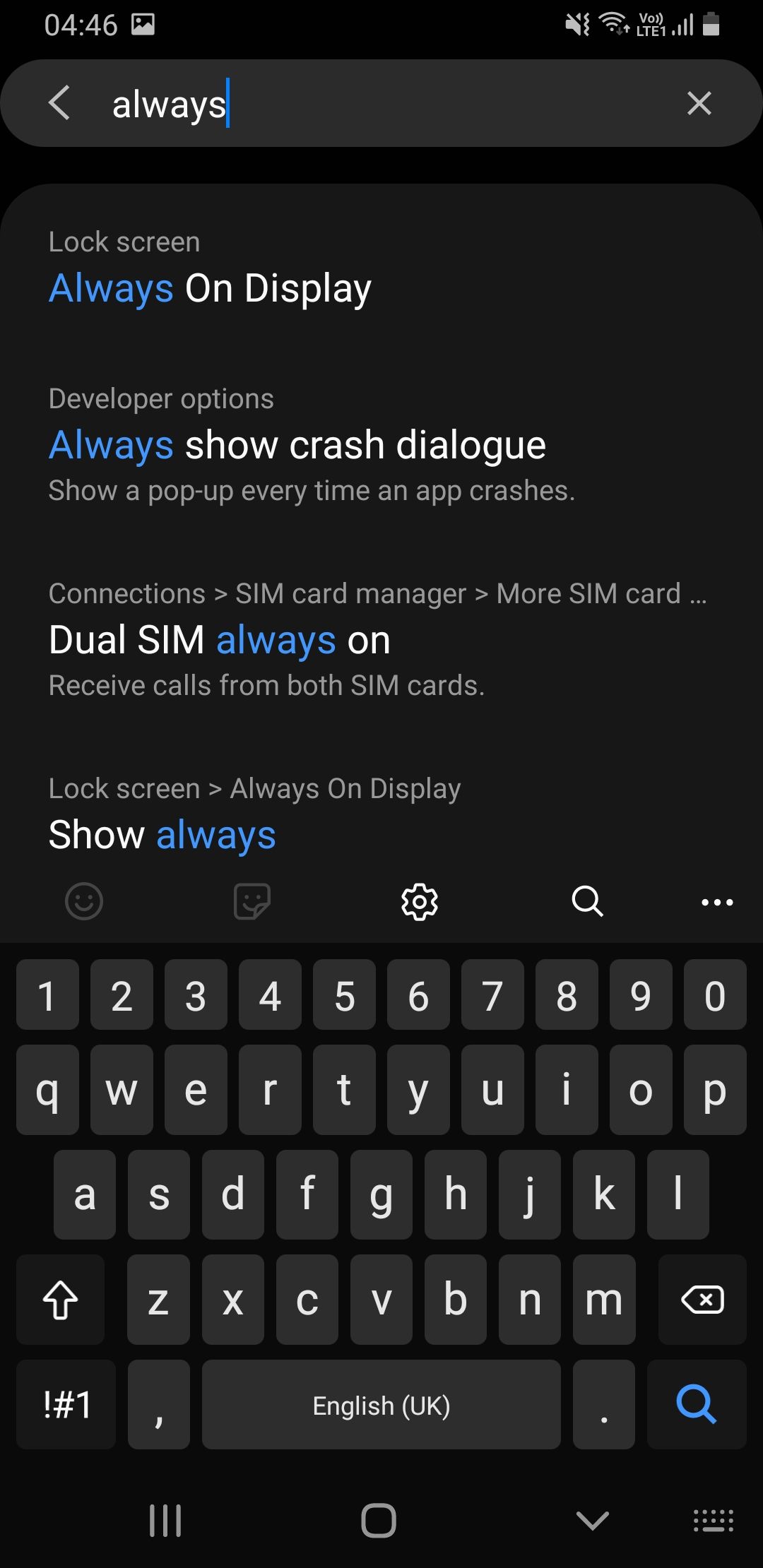This is a detailed screenshot of a smartphone display taken at 4:46 o'clock. The top of the screen features the current time. Below that, there's a navigation bar with a left-facing back arrow and an 'X' button for closing the current view. The screen shows options for various settings including 'Always on Top', 'Lock Screen', 'Always on Display', and 'Developer Options'. Additional options visible include settings for 'Always Show Crash Dialog', which prompts a popup every time an app crashes, and 'Connections', including 'SIM Card Manager' with features for managing multiple SIM cards, such as 'Dual SIM' and the ability to always receive calls from both SIM cards.

The lower portion of the screenshot reveals the on-screen keyboard. The background is black, creating a high-contrast display, and the keys are also black with white letters. The keyboard includes an up arrow key, and the space key is labeled "English (UK)". A blue magnifying glass icon is located in the bottom-right corner of the keyboard, indicating a search function.